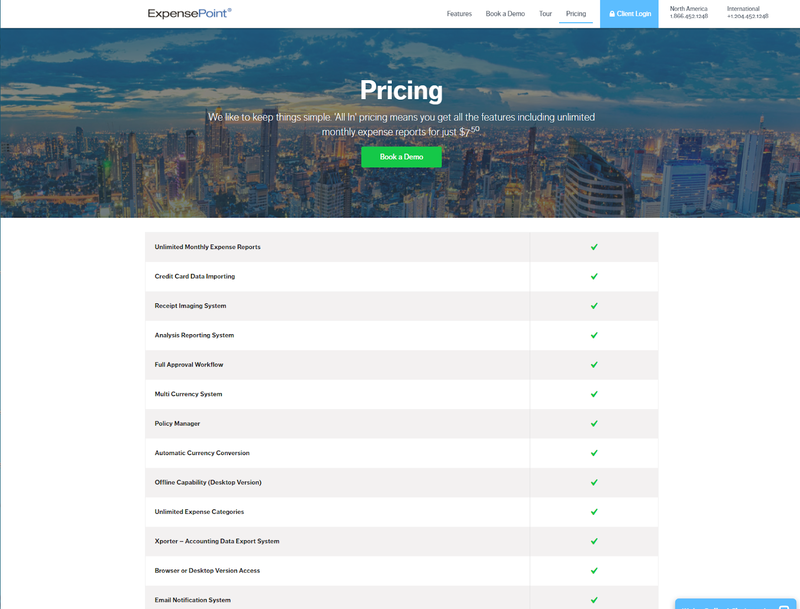This image is a screenshot of a company's website titled "Expense Point." At the top of the webpage, there is a navigation bar containing several dropdown menu options. From left to right, the options are: "Features," "Book a Demo," "Tool Tour," and "Pricing." Other elements on the top right corner include links labeled "Client Login," "North America," and "International," along with respective phone numbers for North American and international inquiries.

The central portion of the webpage features an image of a cityscape under cloudy skies. Overlaying this background is bold white text that reads "Pricing." Beneath this headline, additional text states, "We like to keep things simple. All-in pricing means you get all the features including unlimited monthly expense reports for just $7.50." Directly below this text is a grey button labeled "Book a Demo."

Towards the bottom of the image, there are multiple clickable sections indicated by green check marks aligned vertically, offering more detailed information as the user scrolls down the page.

Overall, the web layout is clean, professional, and user-friendly, designed to provide comprehensive information about the company's pricing and features, with easy navigation options for prospective clients.